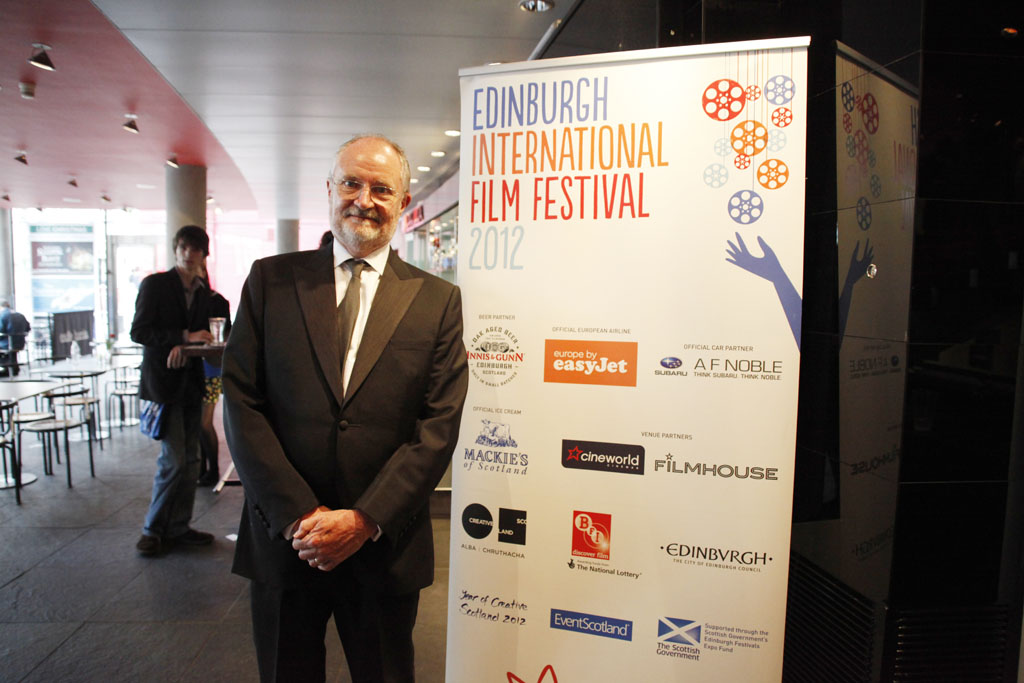This is a detailed color photo of a bald man with fine-rimmed glasses and a closely-shaved goatee. He is wearing a dark black suit paired with a white button-up shirt and a lighter black tie. The backdrop features a sign for the Edinburgh International Film Festival, adorned with film reels in red, orange, and purple, along with a purple arm extending below them. The text "Edinburgh" appears in blue, "International" in orange, and "Film Festival" in red, with "2012" written beneath in light blue letters, followed by logos of various businesses. The man stands in what looks like a cafeteria or food court area. Behind him, there are several people, one of whom appears to hold a tray of food with hamburgers and drinks. The backdrop includes small tables with chairs and stools, and the ceiling is decorated in white and red.